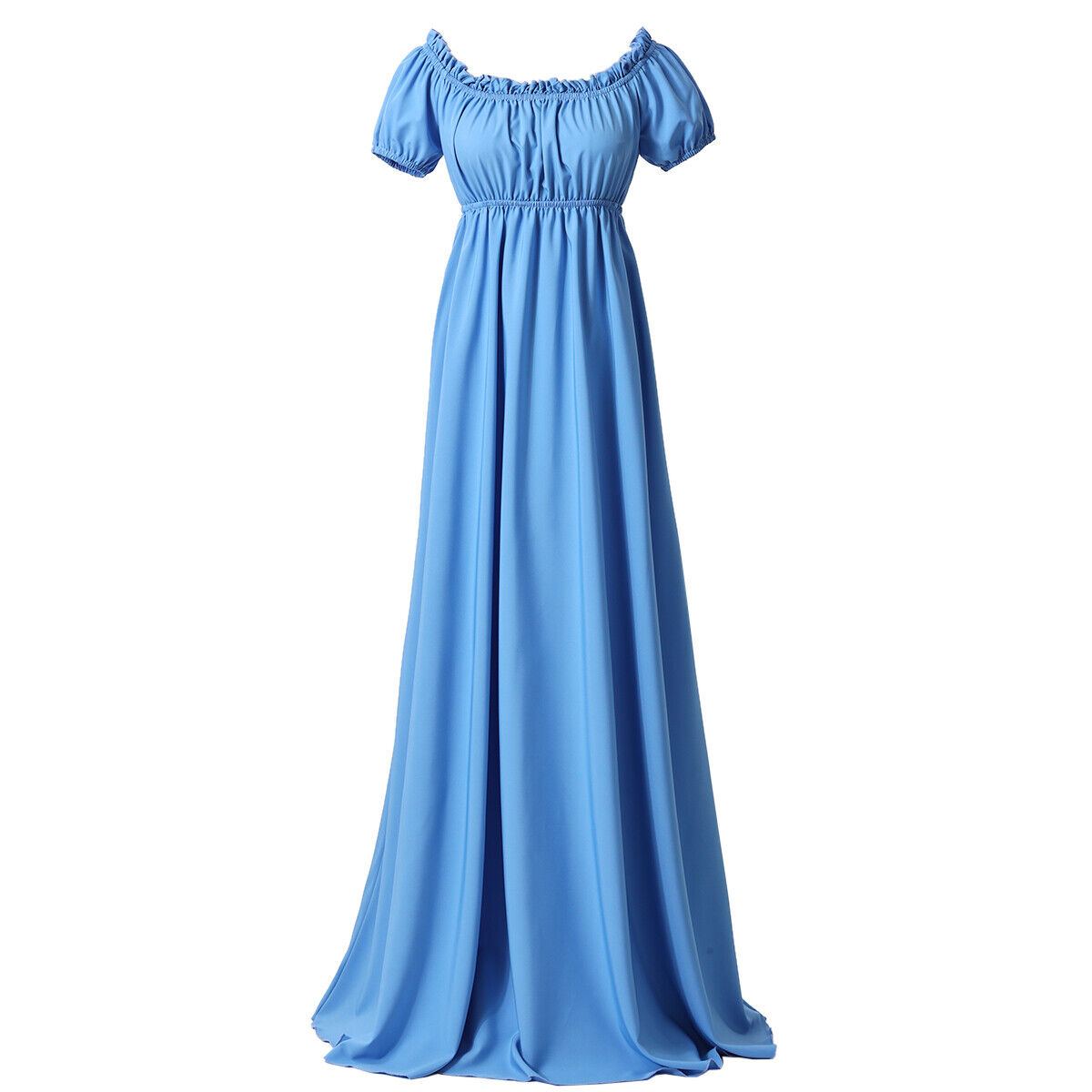This image features a modern interpretation of a late 1700s to early 1800s empire-waist dress, rendered in a contemporary powder blue color. The dress is displayed against a solid white background, highlighting its elegant simplicity. It has a high empire waist, accentuating the area just under the bust, with an elastic band that cinches and defines the upper mid-length breastbone area. The neckline is modestly high yet wide, suggesting it could rest off the shoulders, adorned with a blue ruffle-like texture for added detail. Short sleeves with elastic bands provide a snug fit around the arms, enhancing its refined structure. The dress flows gracefully to the floor, draping in multiple soft, silky layers that suggest a cotton fabric, creating a full, elegant silhouette. This versatile piece, devoid of any embellishments or rhinestones, combines historical inspiration with modern style, making it suitable for contemporary formal occasions.